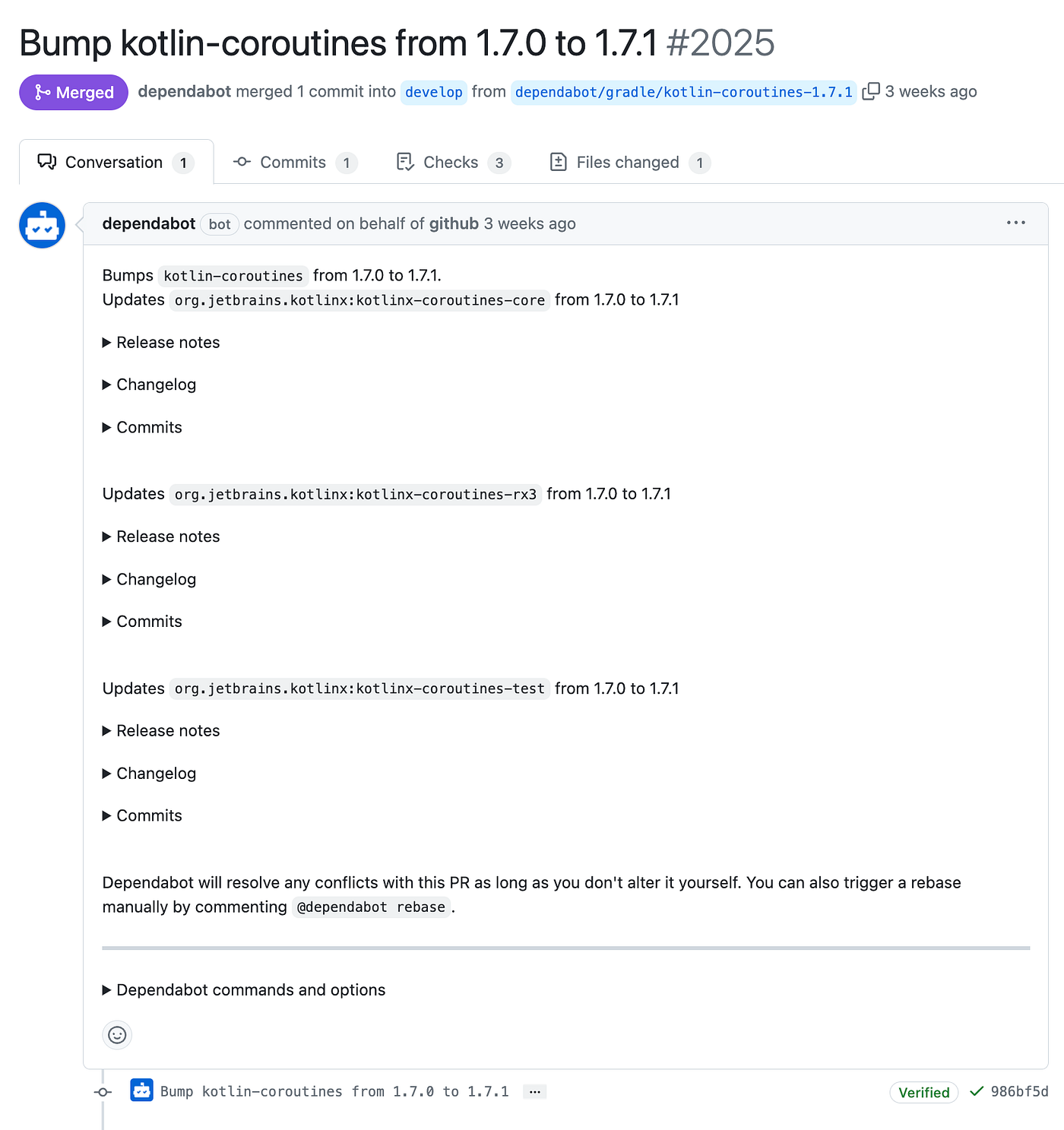The image displays a GitHub interface detailing a recently merged pull request. At the top of the image, a header states "Bump Kotlin-coroutines from 1.7.0 to 1.7.1 #2025." Below this, on the left side, there is a purple "Merged" status bubble indicating the successful integration of changes. The text beneath reads, "dependabot merged 1 commit into develop from dependabot/gradle/kotlin-coroutines-1.7.1 three weeks ago."

Further down, four interactive tabs are visible. The selected "Conversation" tab shows a comment from Dependabot on behalf of GitHub, including release notes, a changelog, and updates. Adjacent tabs labeled "Commits," "Checks," and "Files changed" display notification badges indicating activity: one notification for "Commits," three for "Checks," and one for "Files changed."

At the bottom right corner of the image, a green and white "Verified" badge confirms the authenticity of the merged pull request.